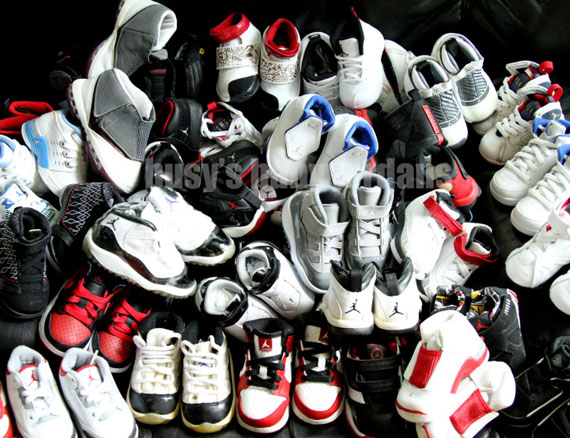This photograph showcases a colorful, jumbled pile of baby and toddler sneakers, mainly Baby Jordans, set against a black background. The shoes vary widely in color, including shades of white, black, red, yellow, gray, and sky blue. Each pair is carefully set, yet piled on top of one another, creating a vibrant, chaotic scene. Many of the shoes feature the iconic Michael Jordan logo, depicting a figure mid-dunk with legs spread. Various styles are represented, such as Velcro, slip-ons, and those with shoelaces. In the center of the image, though somewhat faded, the words "Busy's Baby Jordans" can be discerned, hinting at the branding and focus on these tiny athletic shoes.